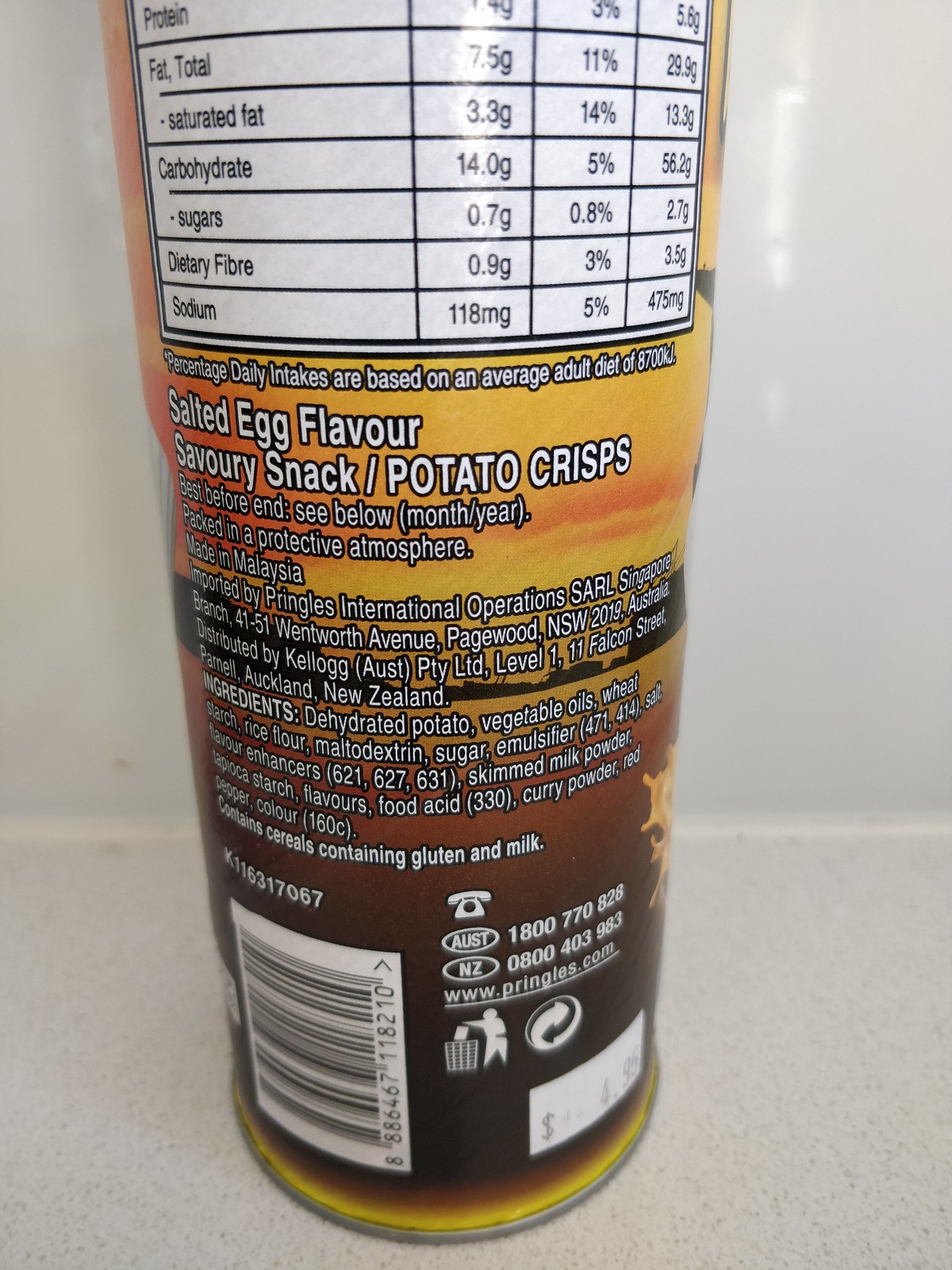The image showcases the back of a cylindrical food container, adorned with a yellow-orange logo. The visible portion of the label reveals part of the nutrition facts, starting from the total fat content, with the information on protein partially cut off above. Additionally, the label identifies the product as salted egg-flavored savory snacks/potato crisps. The packaging also includes a manufacturer address located in Auckland, New Zealand, indicating its origin.